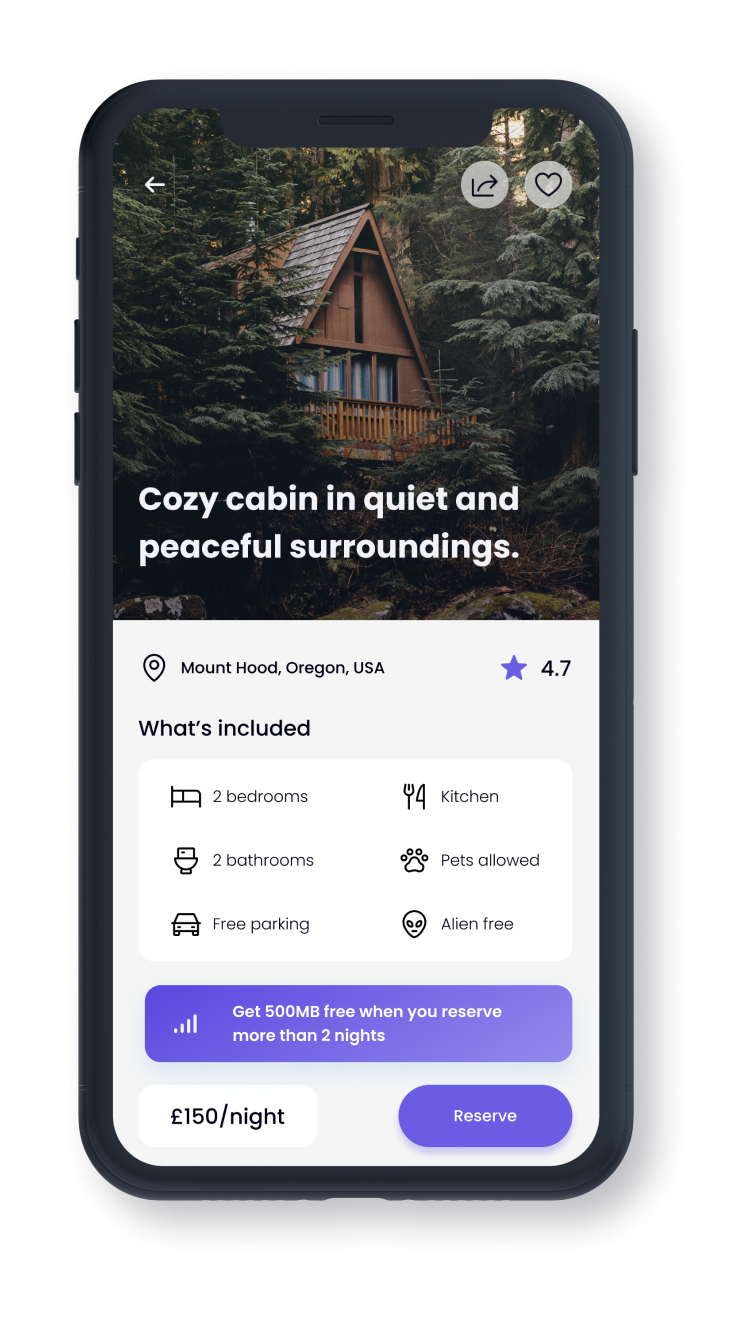In the image, there is a website screenshot displayed on a black phone with a white background. The website appears to be a listing on Airbnb. At the top of the screen, there is a white back arrow and two icons—a hat and a share symbol—both in black ink with a gray circular background.

The main content of the website shows a photograph of a rustic wooden house surrounded by lush greenery. Accompanying the image is a description reading "Cozy cabin in quiet and peaceful surroundings." The listing specifies the location as Mount Hood, Oregon, USA, and indicates a rating of 4.7 stars with a purple star icon.

Additional information provided includes amenities such as a bedroom, bathroom, free parking, kitchen, and pet allowances. Text written in white on a purple background states the cost at £450 per night. There is also a purple "Reserve" button visible.